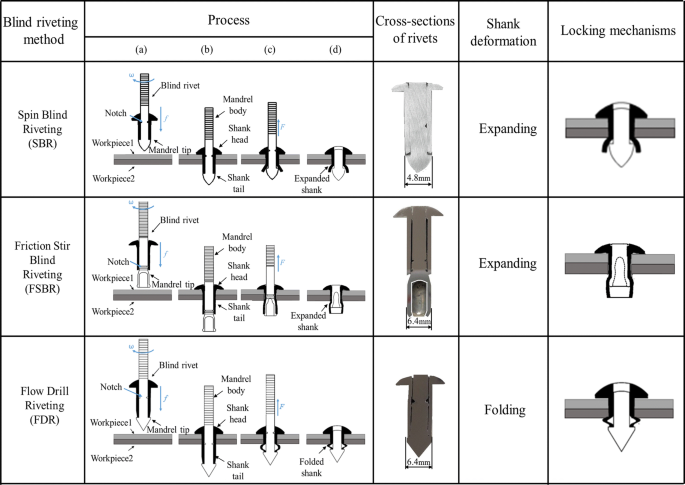This is a detailed horizontal rectangular table on a white background that explains various methods and mechanisms of blind riveting focusing on three different kinds of rivets: two expanding and one folding. The top row lists the types of blind rivets—Spin Blind Riveting, Friction Stir Blind Riveting, and Flow Drill Riveting, each accompanied by illustrations and descriptions. The middle section is dedicated to process diagrams showing how each rivet type is inserted and fastened, providing cross-sectional views of the rivets, the deformation of the shank, and step-by-step insertion details. The bottom row details the locking mechanisms for each rivet type, indicating how the expanded or folded materials secure the joint. The overall layout helps in understanding the full process of blind riveting, from the insertion to the securing of materials.